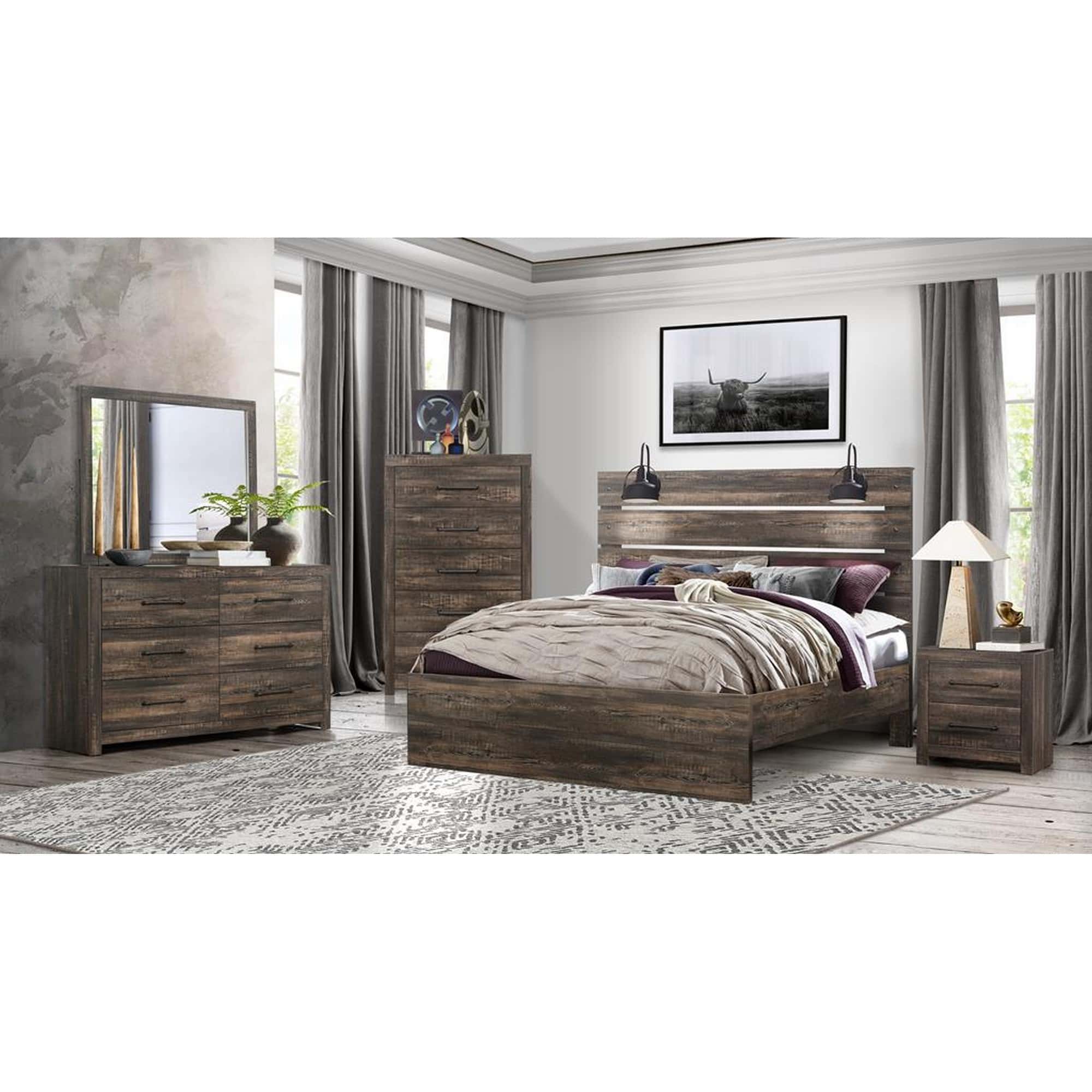This photograph captures a meticulously designed, professionally staged bedroom with a blend of modern and rustic elements. The room features light grey walls adorned with a painting of a cattle with long horns framed in black above a king-size wooden bed that is brown in color. The bed is dressed in brown bed sheets, layered with multiple pillows, cushions, and a quilt. Below the bed lies a grey and white patterned rug, accentuating the wooden plank flooring.

On each side of the bed, there are wooden nightstands with drawers—one on the right side hosts a lamp with a lampshade and an additional small artifact, while the left side has a similar setup. A large cabinet with multiple drawers sits to one side of the room, topped with various artifacts and bowls, and beside a large mirror.

Towards the corners of the room, additional wooden cabinets are noticeable, one of which doubles as a dressing table adorned with a flower vase and other decorative items. Large glass windows with dark grey curtains flank the room, ensuring privacy while complementing the overall color scheme. The ceiling features a white and grey border that adds a sophisticated touch to the space.